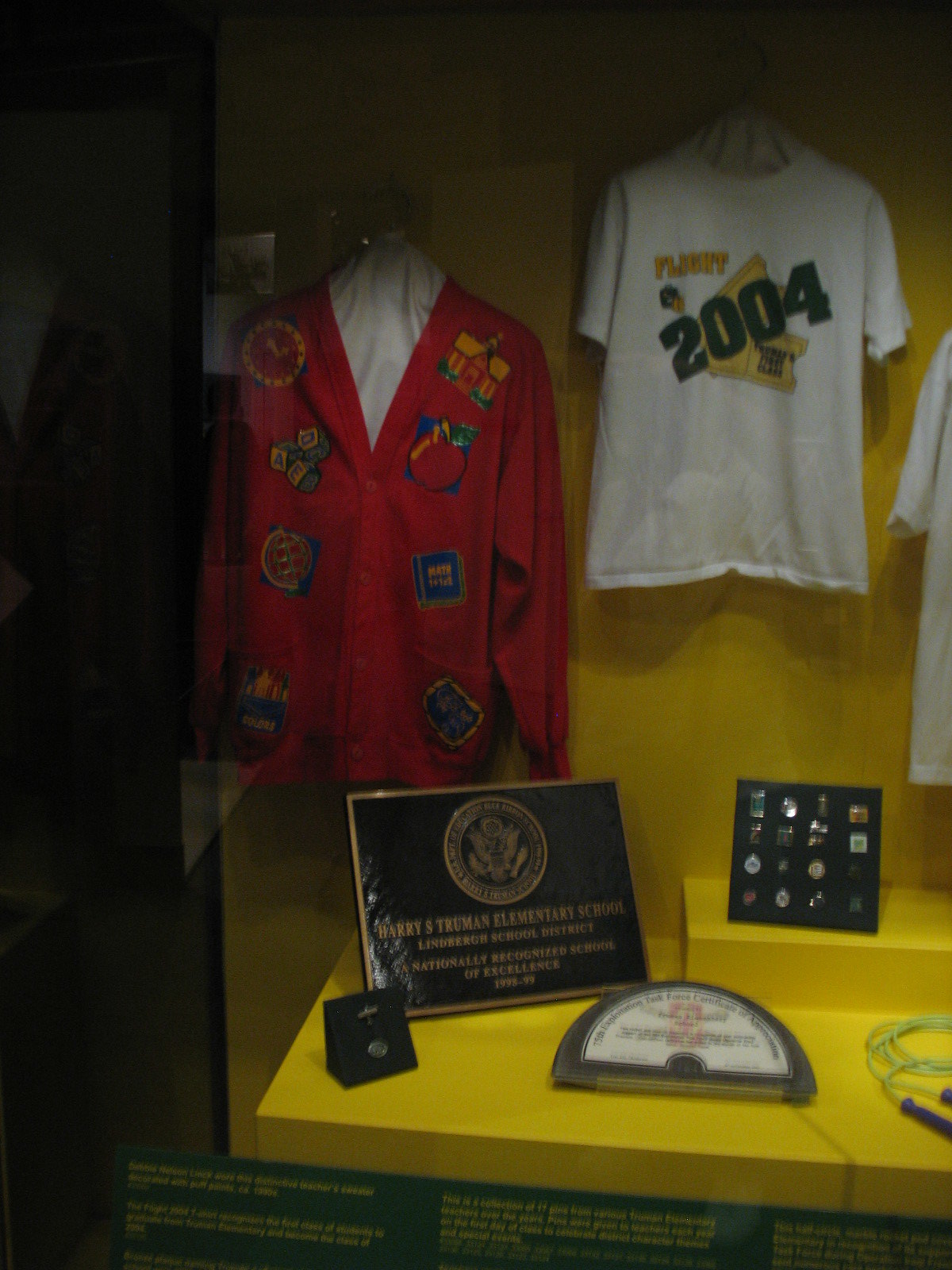Displayed within the museum is a carefully curated exhibit dedicated to the Harry S. Truman Elementary School, part of the Lindbergh School District, recognized nationally as a School of Excellence during the 1998-1999 period. Prominently featured is a federally affixed seal from the Department of Education, establishing the school's esteemed status.

In the exhibition is a Certificate of Appreciation from the 75th Exploitation Task Force, hinting at a broader historical context connecting the school community. The display includes a nostalgic, visual array of school memorabilia: a jump rope, various awards, and a distinctive pin collection. One noteworthy garment on display is a sweater adorned with puff paints, worn by Debbie Nelson Link, a beloved teacher, circa the 1990s.

The display showcases a collection of 17 pins, each representing a unique artifact from different Truman Elementary teachers throughout the years. These pins were ceremoniously bestowed each year on the first day of school, symbolizing distinct character themes and special events, capturing the essence and spirit of the school community.